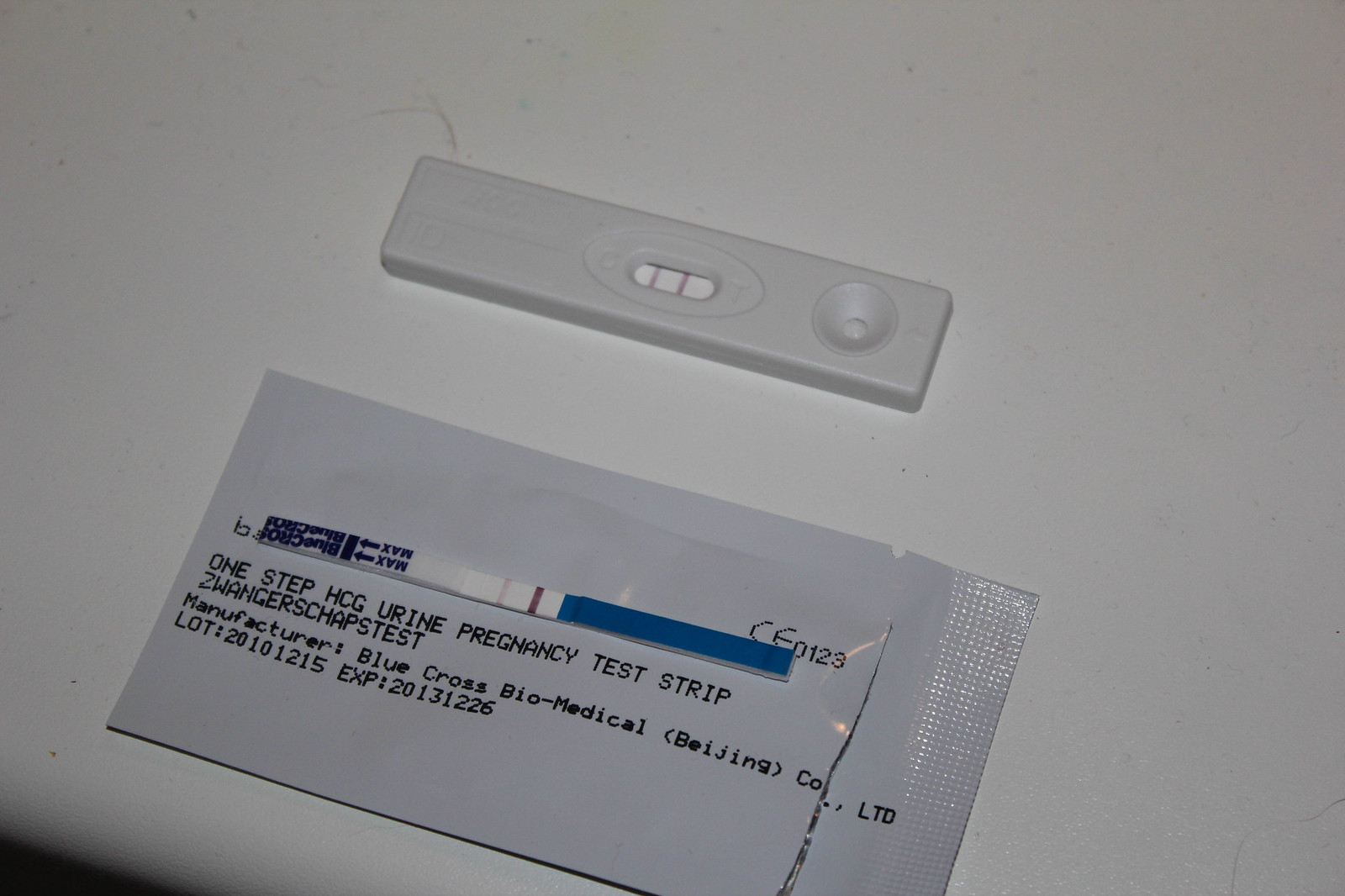The image displays a home pregnancy test kit consisting of several components designed to test for pregnancy using urine. Central to the kit is a long, narrow, sealed blue and white strip featuring two lines: one dark brown and the other tan. The strip is labeled as a "One Step HCG Urine Pregnancy Test Strip" and is manufactured by Blue Cross Biomedical in Beijing, with an expiration date of February 26, 2031. Additionally, the kit includes an off-white plastic holder shaped rectangularly, designed to cradle the test strip securely. At one end of the strip, there is a small, bowl-like indentation intended to collect the urine sample. The center of the strip contains observation windows that reveal color changes indicating the test result. The entire kit is showcased against a clean, white background, highlighting its components clearly.